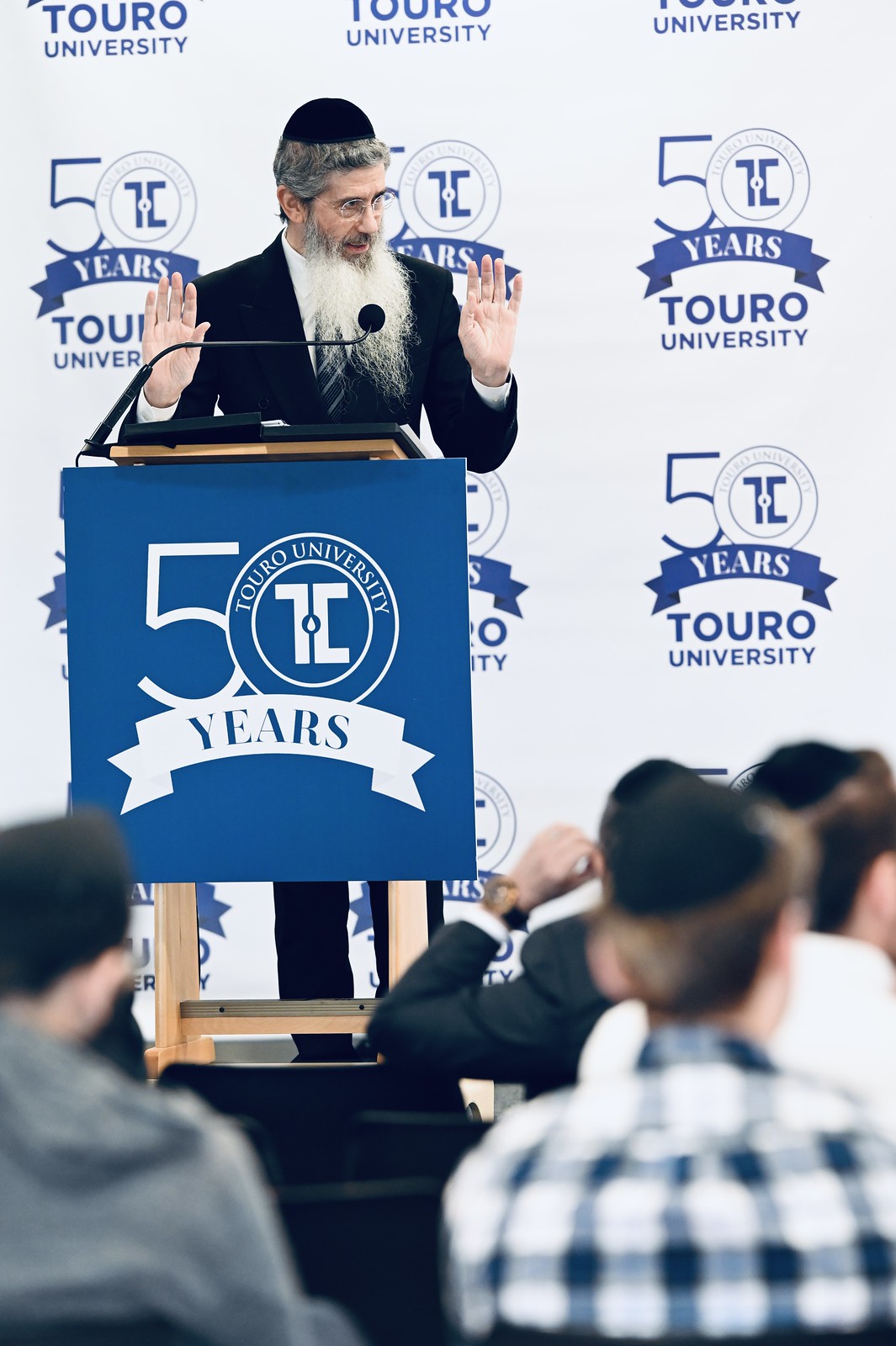In this image, a distinguished Jewish speaker with a substantial, grey-white beard and matching grey hair is addressing an audience from a podium adorned with a blue and white sign that reads "50 years Toro University." This same emblem is also visible on a backdrop banner behind him. He wears a black suit paired with a striped tie in dark hues — possibly navy, green, or blue — and his religious black hat, possibly a kippah or yarmulke, sits atop his head. With his hands raised and palms open, he appears to be emphasizing a point to an audience of six individuals, who are casually dressed but also wearing yarmulkes. The speaker seems highly focused, possibly engaging with an unseen student in the crowd, and the setting indicates a formal event at Toro University.